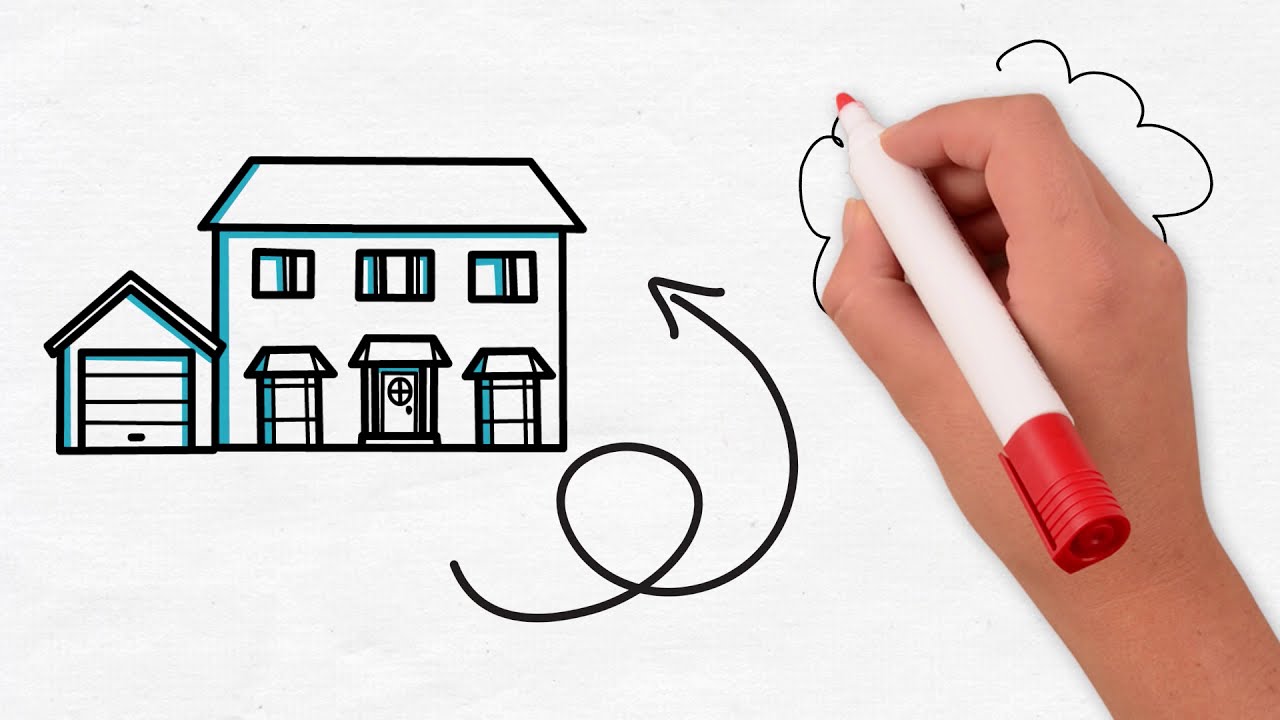The image appears to be a screen grab from an animated informational video. It features a white background with a detailed, cartoon illustration of a standard two-story house featuring a front door, windows, a roof, and an attached garage. Notably, there is a swirly, looped arrow pointing directly to the house. The house is illustrated using black ink with distinctive turquoise shadowing on the windows and door, which includes a circle with a cross design. To the right side of the image, a Caucasian hand is actively drawing with a white marker that has a red cap and nib. This marker is used to draw what appears to be a cloud, although one caption suggested it might be a tree. The scene incorporates colors such as white, turquoise, black, red, and tan. Overall, the image combines elements of real-life video capturing with automated clipart-style animation to convey information visually.